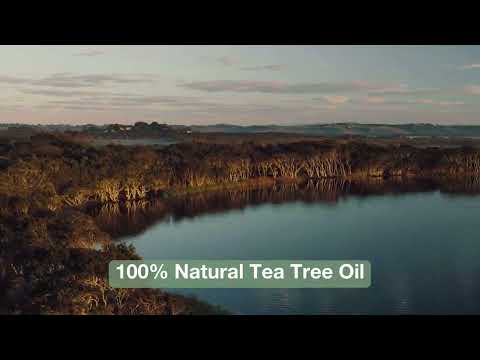This is a video still with a thick black border on the top and bottom, showcasing an aerial view of a serene, tree-lined lake at dusk. The sky is tinged with soft hues of blue, gray, and pink, indicating the sun has recently set, and is adorned with drifting clouds. The lake, illuminated by the faint glow of the evening sky, appears as a light grayish-blue expanse on the right-hand side, while the trees – a diverse mix of light brown, dark green, and dark brownish-yellow tones – wrap consistently around its edge from the left side, encircling the peaceful water. In the distance, the image reveals additional layers of trees and fields, with mountains faintly outlined on the horizon. At the bottom of the screen, there is a green banner overlay with bold white text that reads "100% Natural Tea Tree Oil." The scene seems to be captured from a high vantage point, possibly by a drone, capturing the full extent of this tranquil, natural landscape.